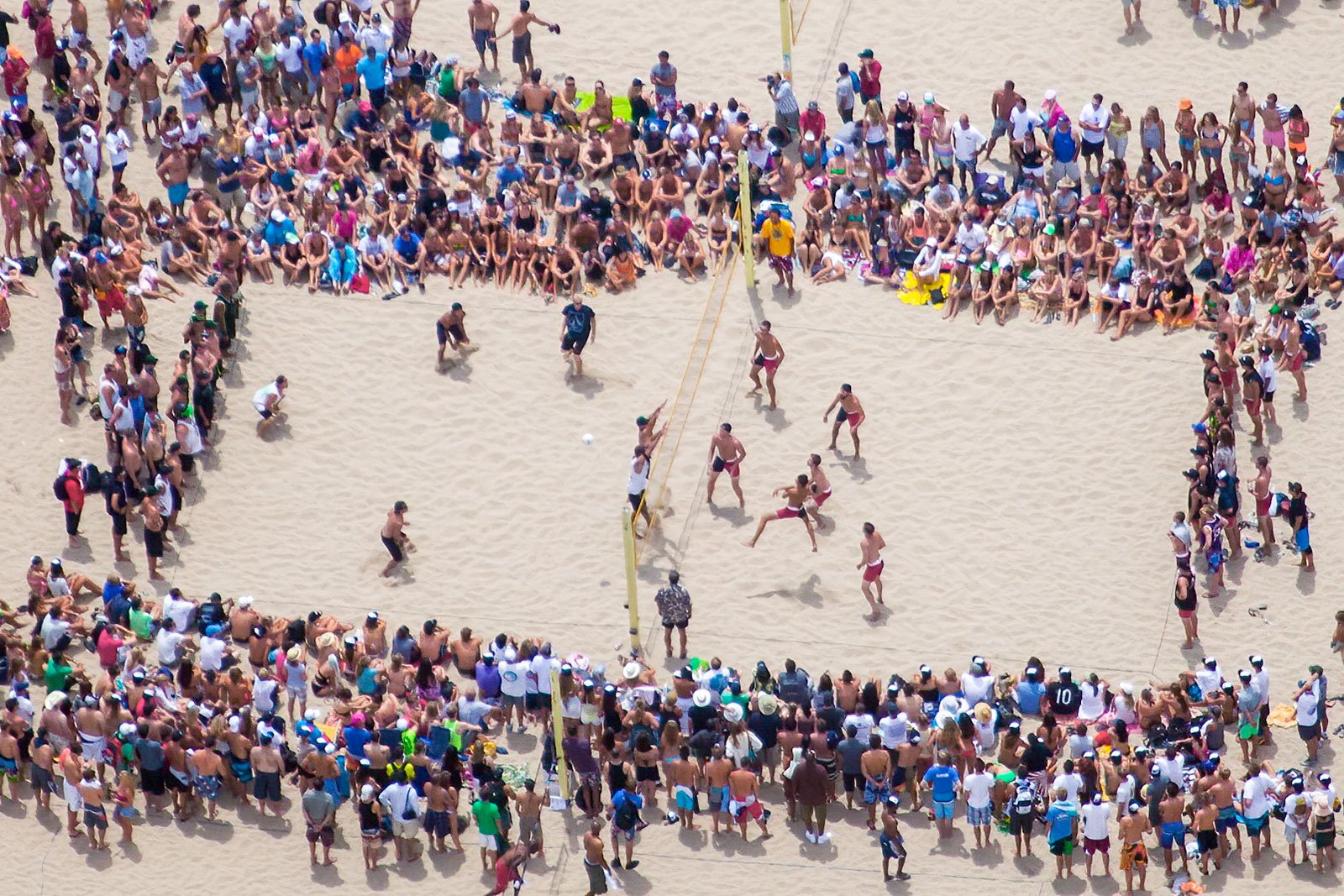This overhead image, taken at a slight angle, vividly captures an intense beach volleyball match on a light beige sandy court. The scene details a six-on-six game with a yellow net prominently dividing the teams. On the right side, a uniformed team of six men in white, red, and black shorts is mid-action, poised to respond to the volleyball that's just come over the net. The left team, comprising six men wearing various black shorts as well as a mix of shirts and bare torsos, is also deeply engaged in the match, with two players up at the net attempting a block and four positioned deeper on the court. Surrounding the court, a vibrant, colorful crowd is seated or standing, mainly densely packed above and below the playing area, creating a striking contrast against the plain light sand. This beach scene is not only lively due to the ongoing match but is also enhanced by the spectators’ varied attire in whites, blues, pinks, and greens. Additionally, visible in the upper part of the photograph is the edge of another volleyball court, hinting at a bustling multi-court volleyball event.